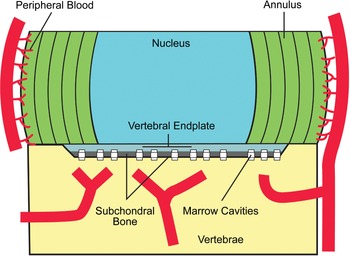This image appears to be a detailed, graphical illustration, likely intended for a medical publication or article. It depicts a cross-sectional view of a part of the human body, with various anatomical structures labeled. The sides of the image feature red, tube-like drawings, representing blood vessels, labeled as "peripheral blood." These tubes transition into a series of green, arc-like shapes labeled "annulus." In the center of the image is a blue, slightly ballooned section marked "nucleus." Below this central section is a light yellow rectangular area containing labels such as "marrow cavities," "vertebrae," and "vertebral end plate," pointing to specific regions within this yellow section. The entire graphic aims to illustrate the relationship between these various parts, potentially focused on structures involved in spinal or vertebral anatomy, as indicated by the presence of vertebrae and marrow cavity labels.